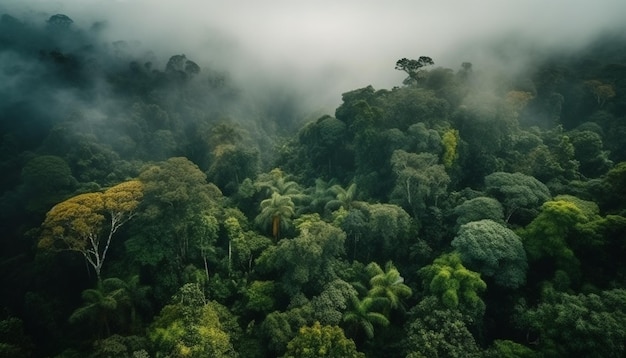This aerial photograph captures a lush, dense rainforest from a high vantage point, providing a top-down view of the vibrant canopy. The forest is characterized by a diverse palette of green shades, ranging from deep, dark green to light green, with the occasional tree appearing almost yellow. The dense tree canopy creates a visual reminiscent of broccoli florets, packed closely together. Some trees exhibit a tropical appearance with branches that flare out, hinting at the varied species residing within the forest.

Additionally, the image features a thick layer of mist or cloud hovering above and weaving through the treetops, adding an ethereal quality to the scene. This fog obscures the background and gives the impression of a misty or cloudy day, enhancing the mystique of the rainforest. The terrain beneath suggests a landscape of hills and valleys, providing subtle depth to the otherwise blanket-like coverage of the trees. Overall, the photograph showcases the rainforest's rich biodiversity and intricate ecosystem from a stunning aerial perspective.